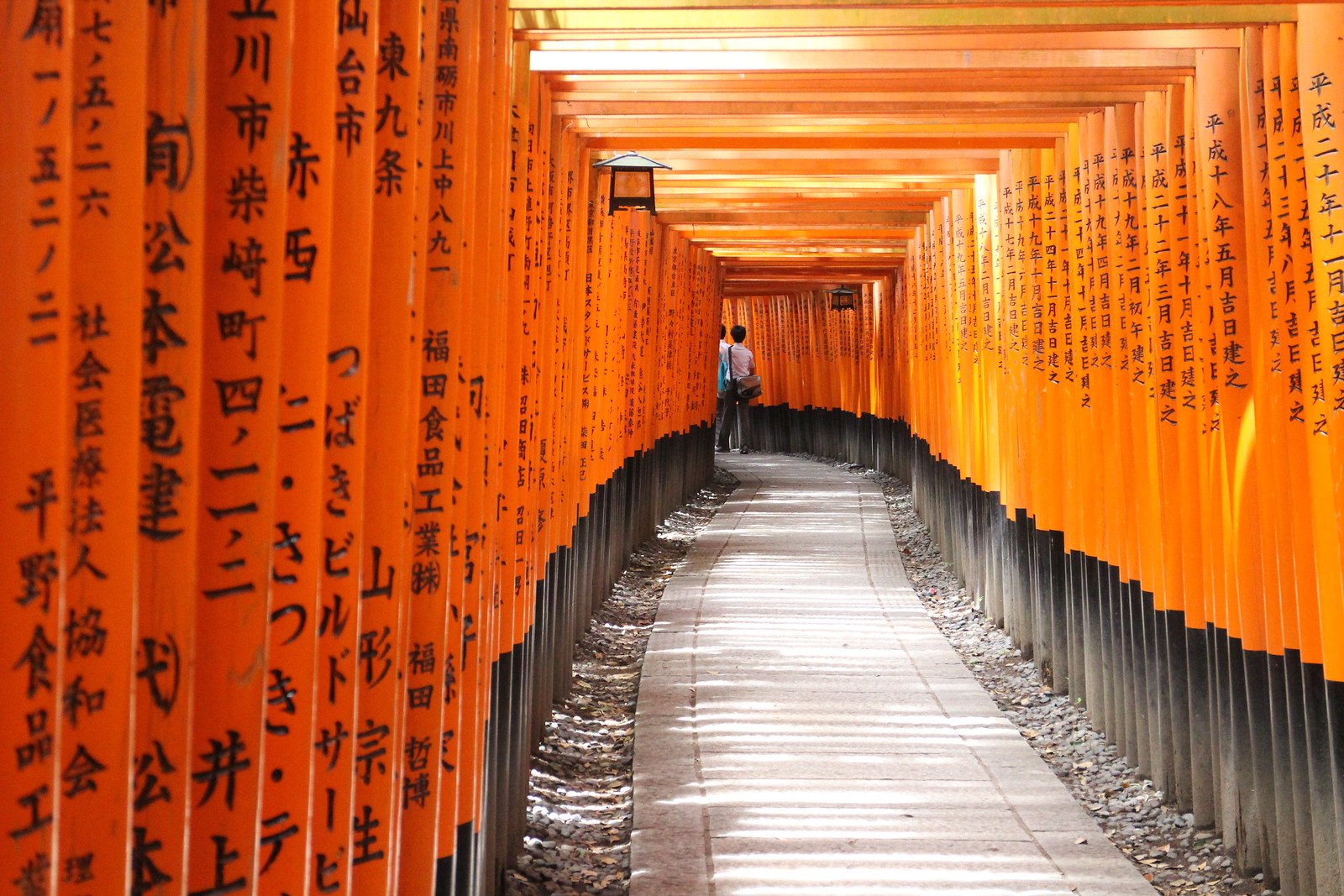This indoor photograph captures a winding concrete pathway that snakes through the center of a dimly lit room, flanked by gray stone or gravel. The pathway is bordered on both sides by a series of orange and black wooden beams or poles, each inscribed with intricate Japanese kanji, creating an almost endless series of personalized messages. Overhead, traditional lanterns are suspended from a wooden or bamboo-style roof, casting a warm glow on the scene below. The distinct combination of the orange wood, black accents, and gray concrete gives the pathway a uniquely vibrant yet subdued ambiance. At the far end of the path, a couple stands; a woman holding a handbag and a person beside her, partially concealed in shadow, identifiable only by their bright aqua-blue jacket.